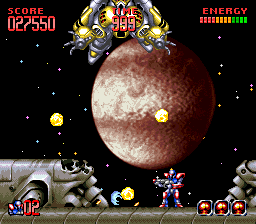Screenshot of a retro side-scrolling game with pixel graphics. The scene is set in outer space, featuring a black backdrop dotted with multicolored specks in blue, pink, and yellow, simulating stars. Dominating the center is a large planet resembling Mars, with a burnt red and brown hue. 

In the top-left corner, the word "SCORE" is displayed in bold red capital letters, followed by the number "027550" beneath it, written in red with a light red stripe running through the center of the digits. 

At the top-center, a floating creature or machine hovers above the planet, accompanied by the text "TIME" and the number "999" below it. The top-right corner features the word "ENERGY" in red capital letters, with a segmented bar below comprising twelve sections. Four segments are red, four are yellow, and four are green, indicating different levels of energy.

The bottom of the screen shows a platform, typical of side-scrolling games, with the player’s character standing on it. The character is donned in a red and blue spacesuit and holds a laser gun. Scattered around the platform are several yellow mid-sized circles. The bottom-right corner of the screen displays three UI squares, while the bottom-left features the number "02" next to a blue icon.